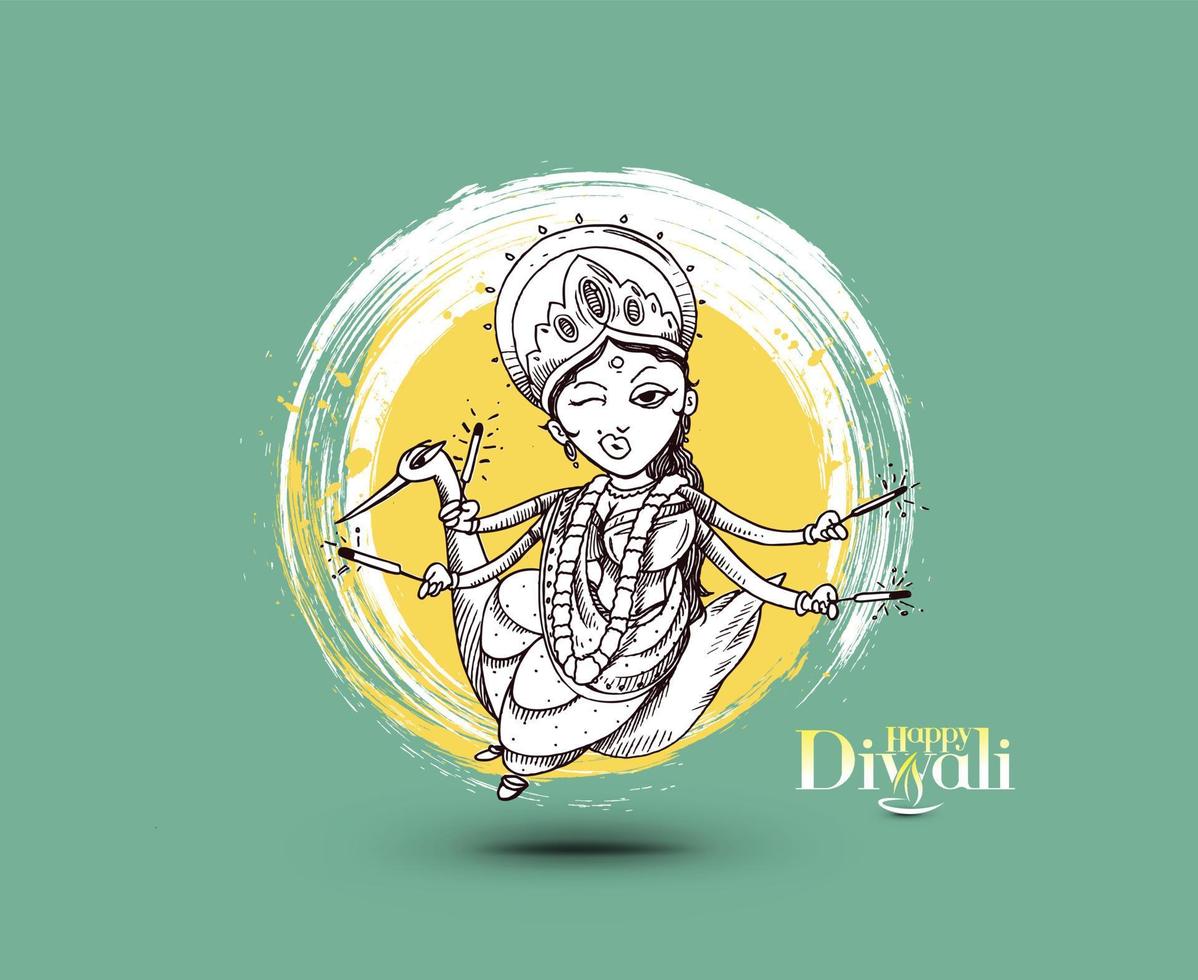The illustration features a black-and-white depiction of a Hindu goddess with long braided hair and four arms, each holding a sparkler. She is wearing traditional Hindu attire, including a crown with three jewels, long robes, bangles, necklaces, and a scarf decoration. She is seated on a peacock, winking happily at the viewer. The background is a mint green, with a central yellow circle surrounded by a white swish circle, resembling a sun or portal. The bottom right corner has the text "Happy Diwali" in yellow and white, with the 'W' stylized as an oil candle, alluding to the Diwali festival.